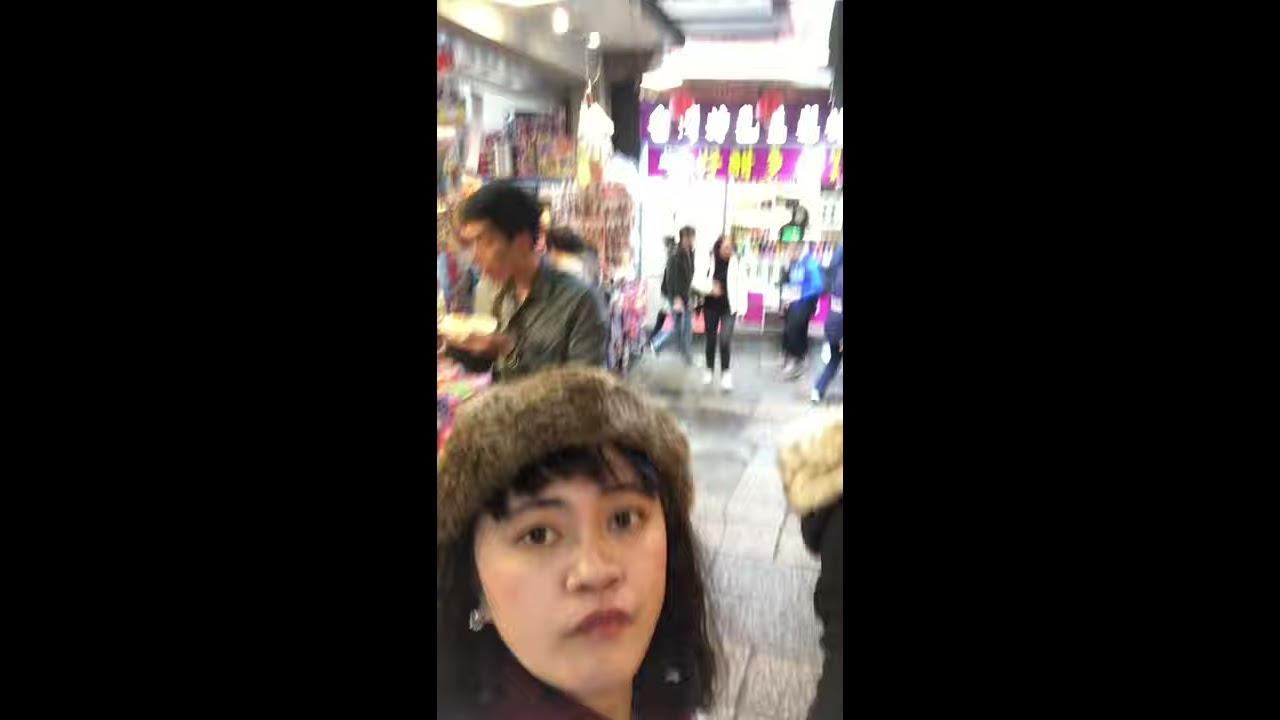In the foreground of this busy and somewhat blurry image, there is an Asian woman with dark hair, dark eyes, and red lips, wearing a fur hat and a single silver earring on her right ear. Her face is clearly visible, but the view cuts off just below her chin. She stands out sharply against the blurry background, which reveals a bustling shop or market with a tiled floor. Behind her is a blurry figure of an Asian man with black hair, possibly holding a plate of food or illuminated by some sort of light. The background is filled with various details, including banners with Asian characters hanging from the ceiling, indicating that this setting is within an Asian community. The scene appears to be quite dynamic, with several people moving around, suggesting a busy market atmosphere. The colors prominent in the image include brown, black, olive, red, pink, silver, yellow, tan, and gray. The market area behind the woman includes what appear to be vendors and windows, lit by a sunny day, further enhancing the lively, bustling environment.